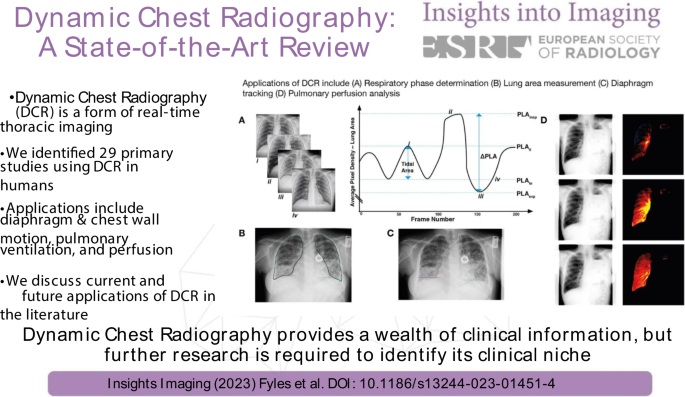The digital image, resembling a presentation slide from a medical website, prominently features the title "Dynamic Chest Radiography: A State-of-the-Art Review" in large purple font at the top. On the top right, beneath the smaller purple text that reads "Insights into Imaging," there's a logo for the European Society of Radiology (ESR). The slide explores Dynamic Chest Radiography (DCR), a form of real-time thoracic imaging discussed through various bullet points on the left side. These points highlight applications such as diaphragm and chest wall motion, pulmonary ventilation, and perfusion, as well as the review and future applications of DCR based on 29 primary human studies. The bottom of the slide states that while DCR provides a wealth of clinical information, further research is needed to establish its clinical niche. Accompanying the text are several images, likely x-rays of chests with highlighted points at their centers, and a chart. Across the bottom, there is a purple bar with black text that reads, "Insights Imaging 2023, Files et al., DOI 10.1186/s13244-023-01451-4."